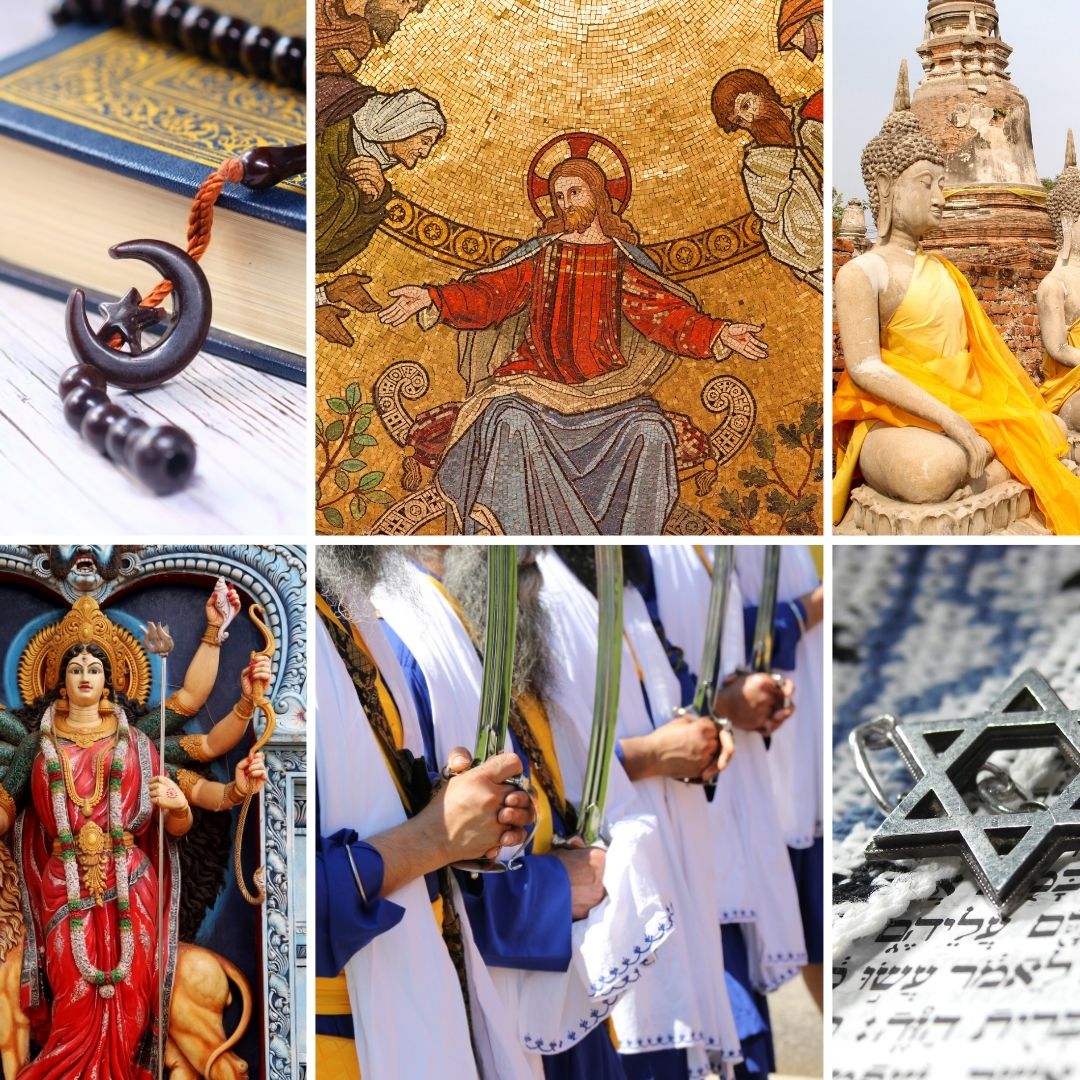The image is a vibrant and detailed collage consisting of six photographs arranged in a grid, each representing different religious imagery. In the top left, there is a crescent moon and star on a heavily ornamented book, symbolizing Islam. The upper center features an intricate mosaic of Jesus sitting in an ornate chair, indicative of Orthodox Christianity. The upper right displays statues adorned in yellow robes, associated with Buddhism. The lower left contains a statue of a Hindu goddess with multiple arms, possibly wearing a flower garland necklace. The bottom center image shows a row of men holding swords, likely representing Sikhism. The bottom right captures the Star of David on a book with modern Hebrew text, symbolizing Judaism.